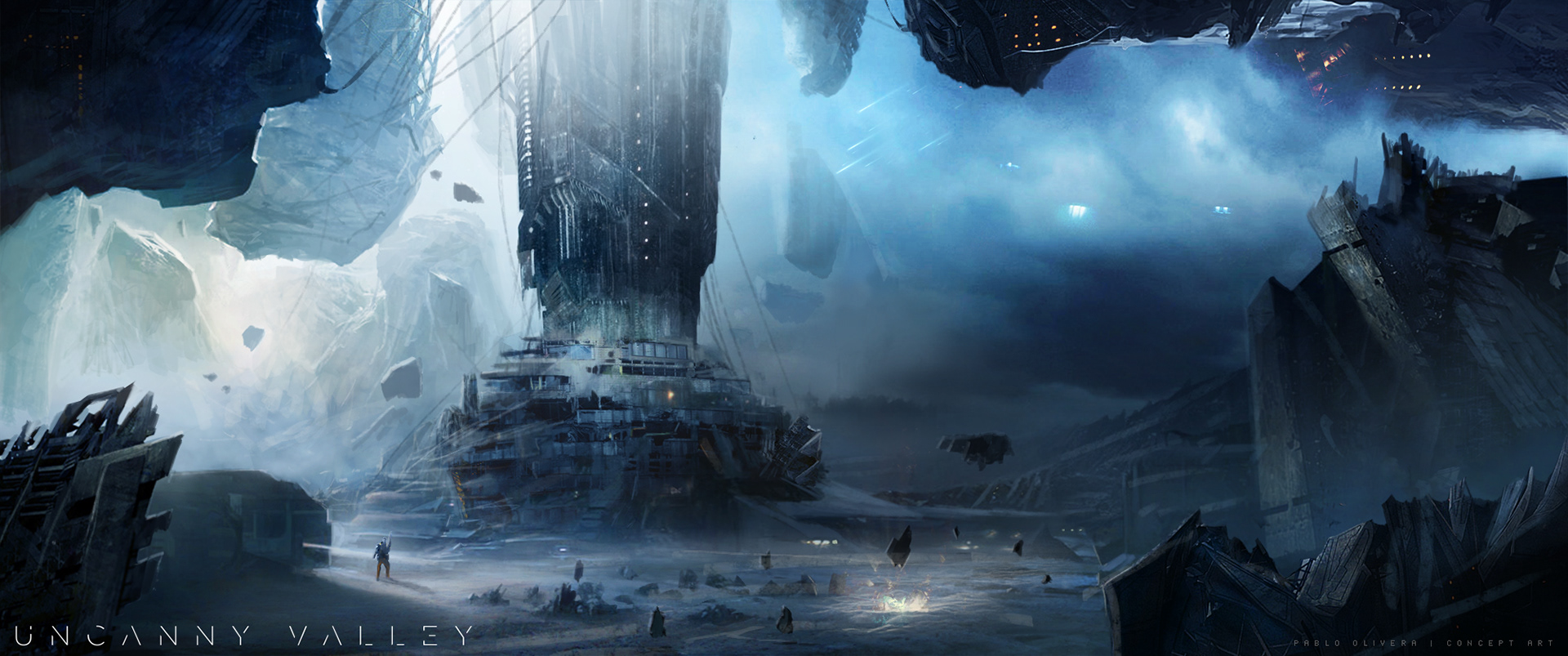The concept art piece titled "Uncanny Valley" by Pablo Oliveri depicts a dramatic and futuristic scene in a widescreen format. At the center of the composition stands a towering, complex structure, possibly a futuristic building or spaceship, featuring multiple layers, segments, and glowing lights that suggest advanced technology. The architecture is detailed and intimidating, with angular parts and jutting sections that reinforce the sci-fi aesthetic of a spaceport or city hub.

The environment surrounding the central structure is equally stark and imposing, characterized by a dark, cave-like setting with floating or falling rocks, hinting at a desolate or post-apocalyptic landscape. The predominant colors are dark charcoal gray, black, and shades of blue, harmonizing the bleak atmosphere. The foreground is shrouded in shadow, while there are bright lights in the background, possibly from an open but dark sky.

Scattered around the massive structure are tiny human figures, dwarfed by the enormity of their surroundings. These figures, possibly armed with guns, accentuate the scale of the scene. Other notable details include wires hanging from the top left, suggesting destruction or disrepair, and orange lights on the top right, possibly indicating windows or technological elements integrated into the rocky formations.

Overall, the image conveys a surreal, possibly dystopian scenario that blends elements of science fiction and advanced civilization with an air of desolation. The impeccable detail and expansive scale of the artwork create a vivid, immersive visual experience, pushing the boundaries of the viewer's imagination.